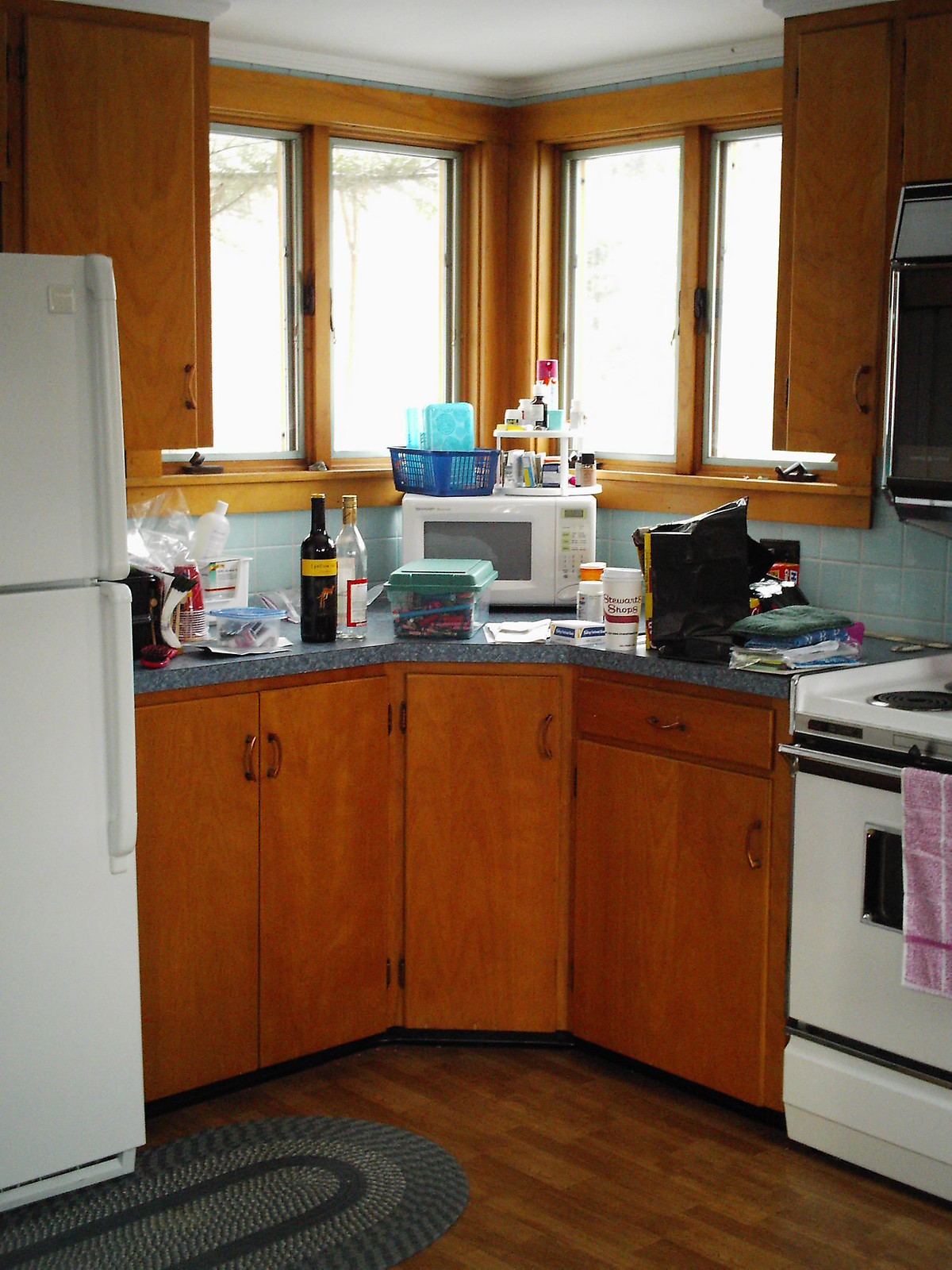The image depicts a cozy corner of a retro kitchen, showcasing a mix of charming, nostalgic elements. The kitchen cabinets, crafted from an orange-hued wood, contribute a warm, rustic feel to the space. The Formica countertop, situated prominently in the corner, adds to the vintage aesthetic. The walls behind the countertop are adorned with light turquoise square tiles, bringing a fresh pop of color to the scene.

On the right side, an older model range is visible, featuring an oven at the bottom and a pullout storage drawer below. The range is equipped with traditional circular electric burners, a hallmark of mid-century design. Above the range, there's an additional built-in unit, which could either be a microwave or a secondary oven, enhancing the kitchen's functionality.

Windows with casement-style cranks are positioned in the corner, enclosed by the same light orange wood as the cabinetry, creating a cohesive look throughout the kitchen. To the left, stands an old-fashioned refrigerator with a freezer compartment on top, distinguished by long vertical handles on the right side.

The floor features a woven oval rug crafted from cotton, adding a touch of homeliness and comfort. The flooring itself is composed of wooden planks, further accentuating the kitchen's warm, vintage charm.